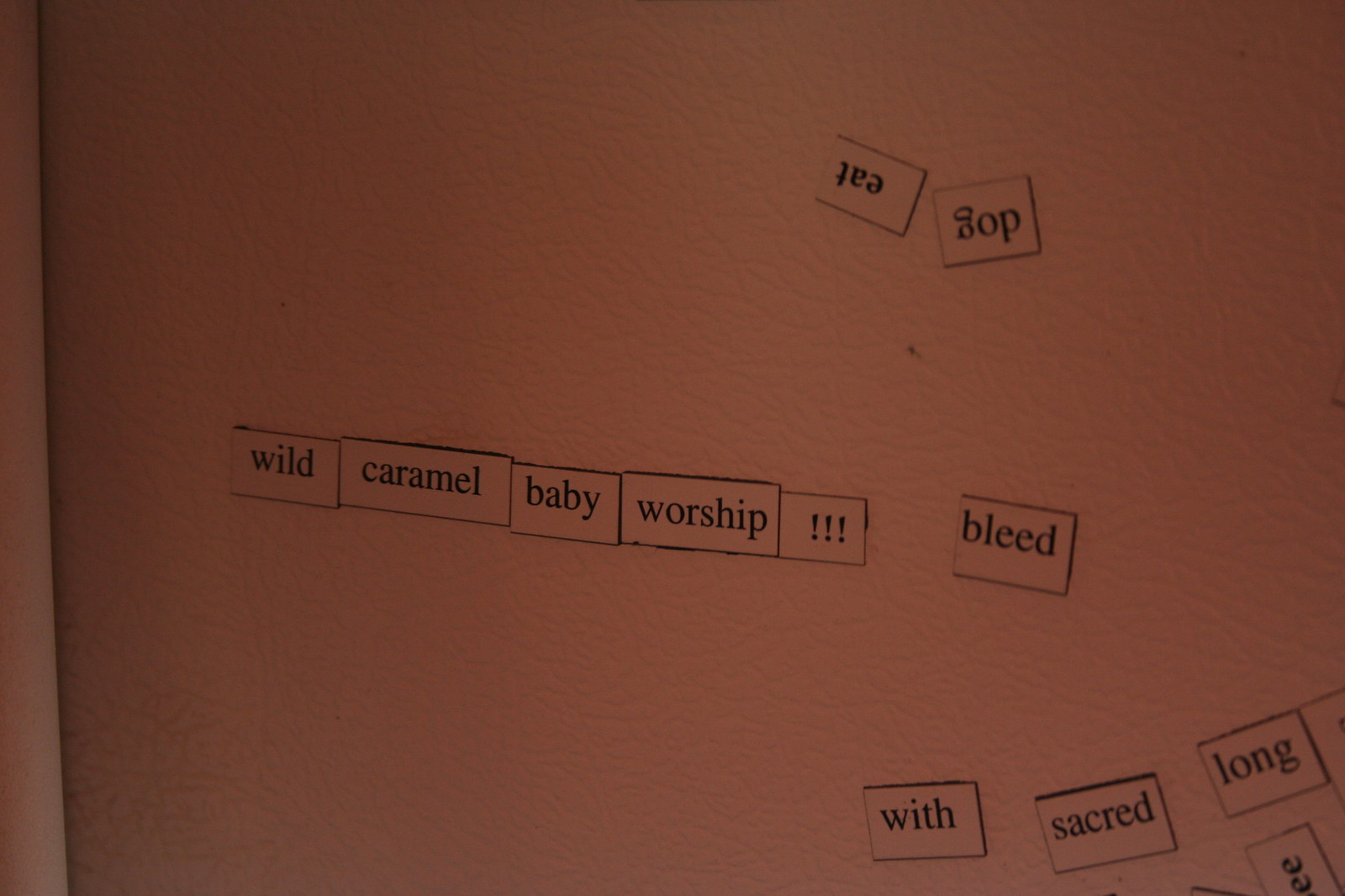This image features a white enamel fridge adorned with magnetic words set against a dark background that transitions from a deep rust color at the top to a lighter pink-red hue in the bottom right corner. Prominently displayed are several black-text-on-white-background word magnets. At the top, two upside-down magnets read "eat" and "dog." Centrally, there's a cluster of magnets forming the phrase "wild caramel baby worship" followed by three exclamation points, with the word "bleed" positioned to the right. In the bottom right-hand corner, the words "wit," "sacred," and "long" appear, with an additional partial magnet showing only two "E's." The overall scene is somber and minimalistic, emphasizing the stark contrast between the dark gradient background and the white, text-filled magnets.